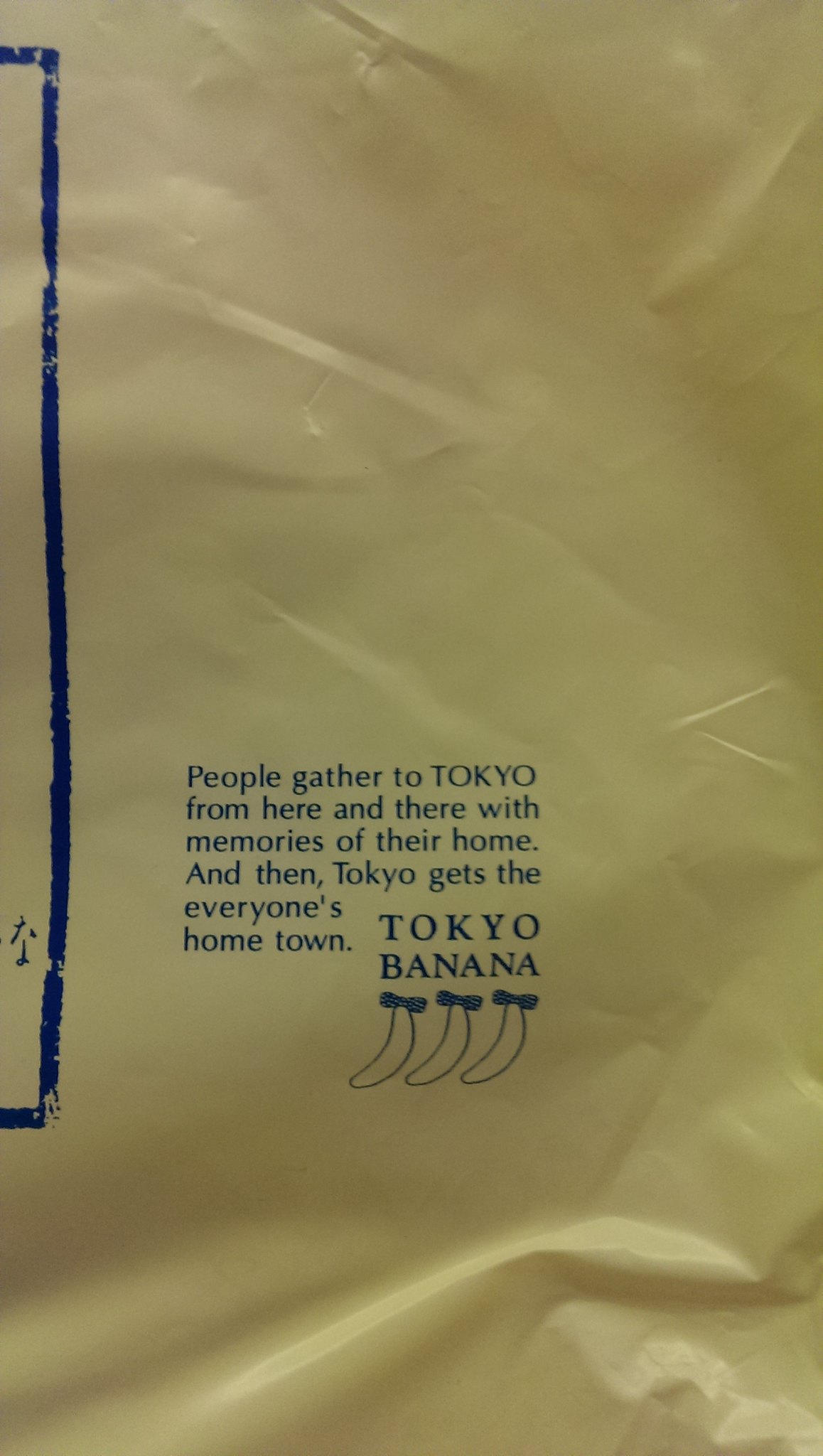The image appears to show a crumpled, tan-colored, possibly plastic or paper material that resembles an old or wrinkled piece of parchment with a hint of goldish yellow hue. On the left side, there is a partial view of a vertical blue rectangle or box. In the center of the image, written in small, blue text, is a message that reads: "People gather to Tokyo from here and there with memories of their home. Then Tokyo becomes everyone's hometown." Towards the lower right of the image, there is a larger text displaying "Tokyo Banana," accompanied by three small, pencil-drawn bananas each adorned with a solid blue bow at the top, where the stem would typically be. This detailed composition suggests that the image might be an advertisement or packaging for the Tokyo Banana brand.